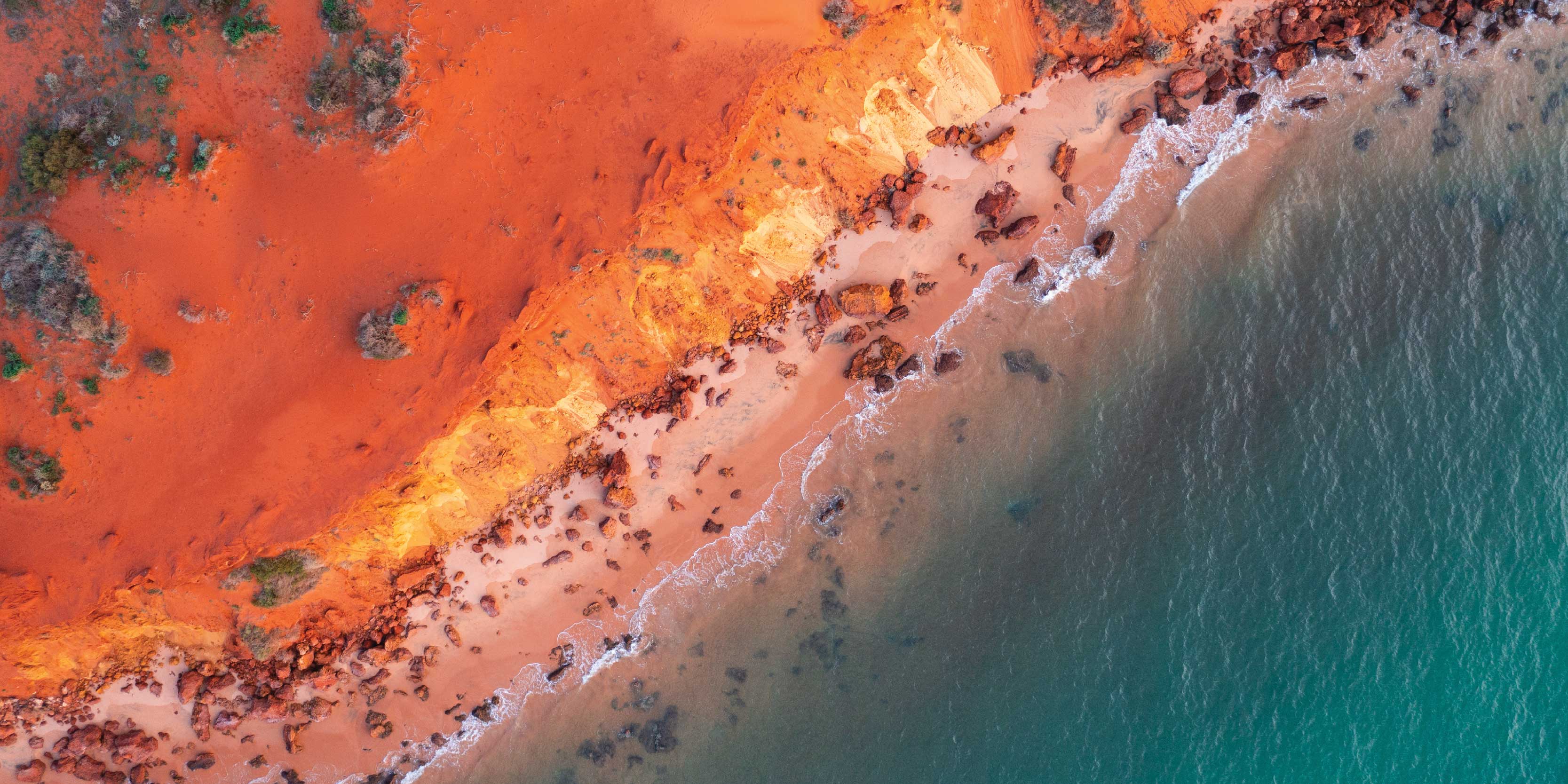This detailed outdoor daytime photograph captures a stunning aerial view of Shark Bay's vibrant shoreline. The rectangular image, approximately 5 to 6 inches wide and 2 to 3 inches high, presents an expansive beach landscape from a directly overhead perspective. The beach, characterized by its bright orange to burnt orange sand, transitions from the upper left corner to the middle of the image. This colorful shore is textured with numerous brownish-orange and gray rocks, some adorned with sparse green foliage. The clear, aqua blue water dominates the lower right portion, moving towards the middle where it meets the shore in a frothy white line of waves. The water's color transitions from a light green near the bottom right corner to darker hues approaching the shoreline. The scene is framed by the contrasting colors of the sand and sea, making the photograph twice as wide as it is tall, an awe-inspiring capture of the natural beauty of Shark Bay.